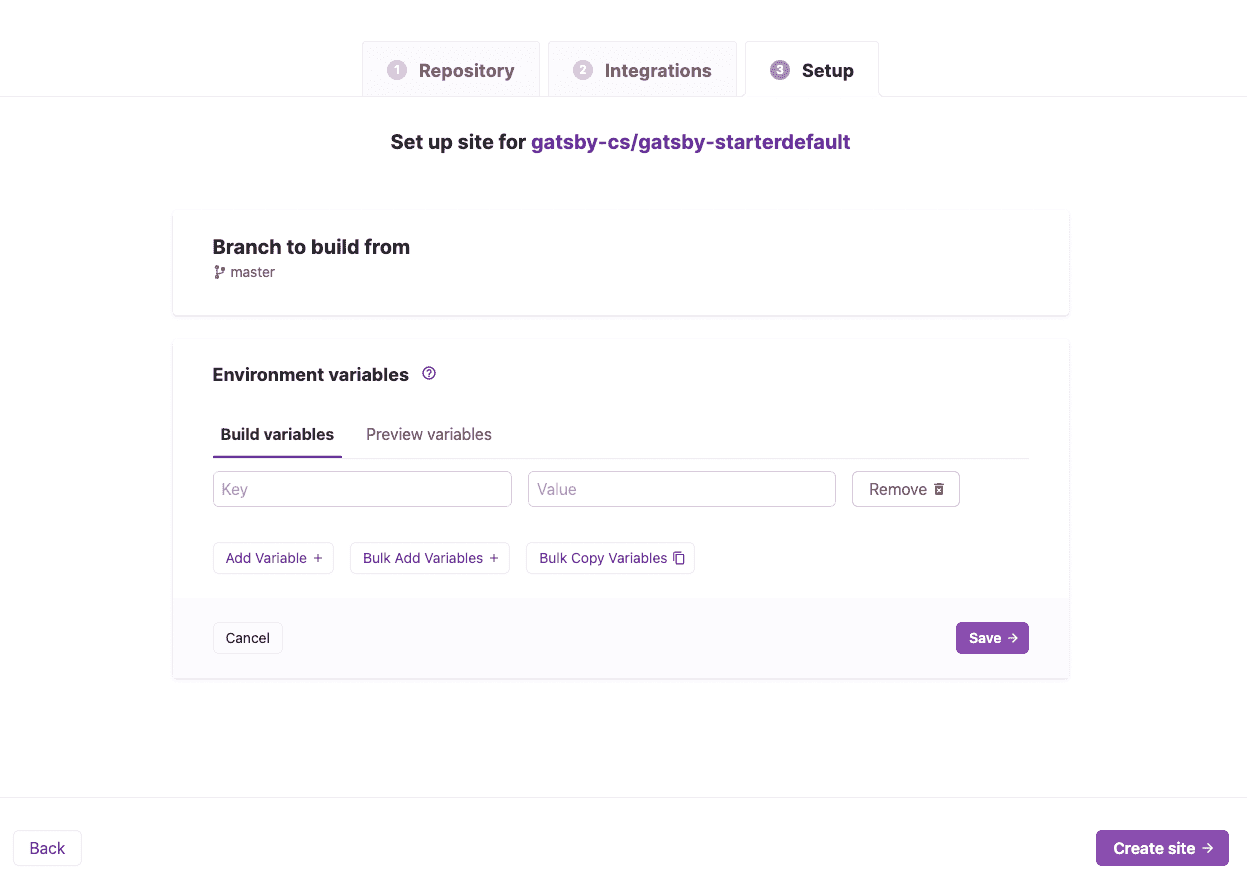This screenshot depicts an interface with three tabs positioned at the top center: "Repository," "Integrations," and "Setup." The "Repository" and "Integrations" tabs appear in a lighter color, indicating that the "Setup" tab is currently selected. Below the tabs, the heading reads "Setup site for gatsby-cs-gatsby-starter-default."

To the left, there is a section titled "Branch to build from," which contains the word "master" in small letters, enclosed within its own box.

Adjacent to this is a larger box labeled "Environment Variables," accompanied by an information icon. Within this box, the "Build Variables" option is selected, while the "Preview Variables" option is present but grayed out. There is a text input row for a key and value pair, flanked by a trash can icon labeled "Remove" for deleting the entry. 

Beneath this row, there are three buttons: "Add Variable +" for adding a new variable, "Bulk Add Variables +" for adding multiple variables simultaneously, and "Bulk Copy Variables" which includes a copy symbol.

In the lower section of the interface, towards the left, is a "Cancel" button. To the right, there's a "Save" button featuring an arrow.

A horizontal line separates this portion from the very bottom of the screen, where two additional buttons are located. On the left is a white "Back" button, and to the right, a purple "Create Site" button adorned with a right-facing arrow.